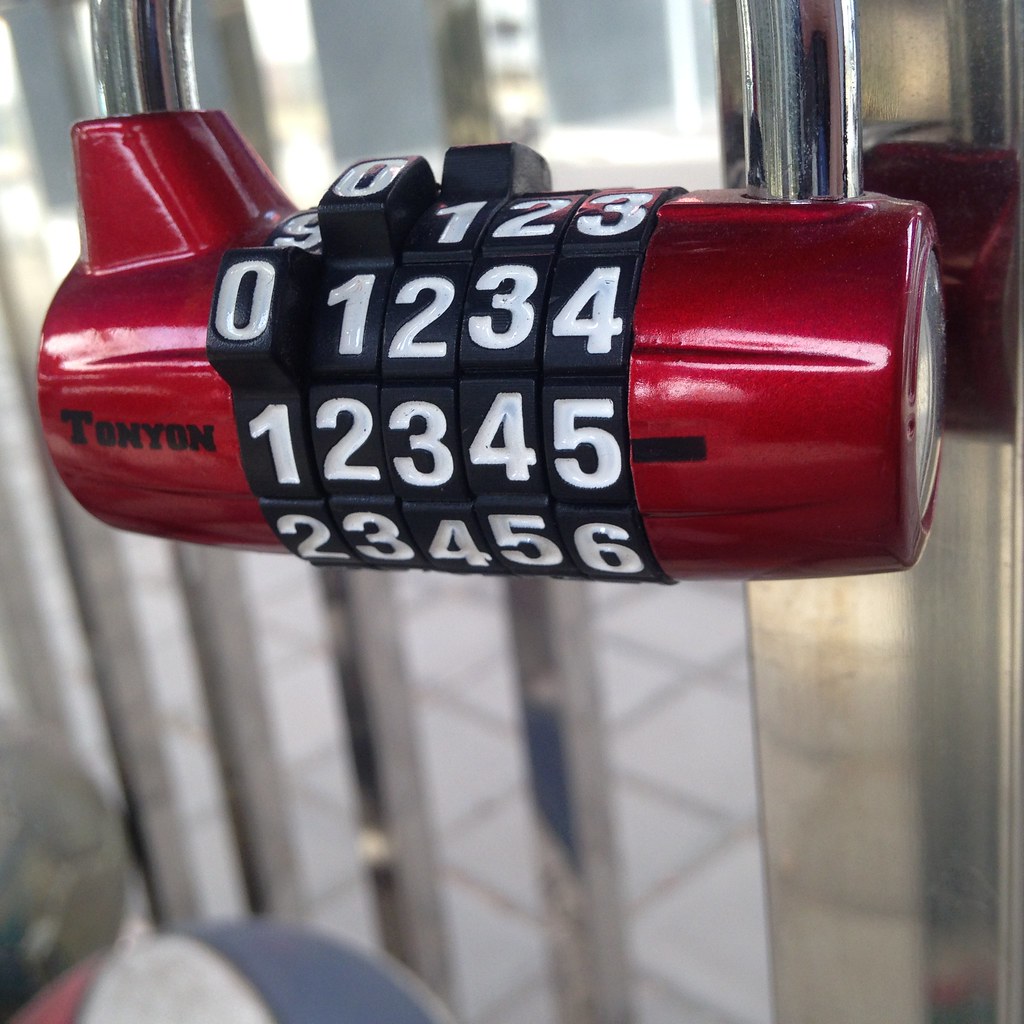The image depicts a detailed close-up of a red metallic padlock with a rounded barrel shape. The padlock's main feature is its combination mechanism, consisting of five black embossed rows featuring white numbers ranging from 0 to 9. Each row has protruding tabs to assist in rotating the numbers to unlock the device. Stamped on the left side of its red base is the black text "TONYON," identifying the manufacturer. The lock is secured against one of the metal poles of a white metal fence. In the out-of-focus background, a door with clear glass window panes framed in silver metallic metal can be faintly seen. The scene suggests the padlock might be used in a gymnasium or similar facility, hinted by the presence of a blurry object resembling a basketball or soccer ball.